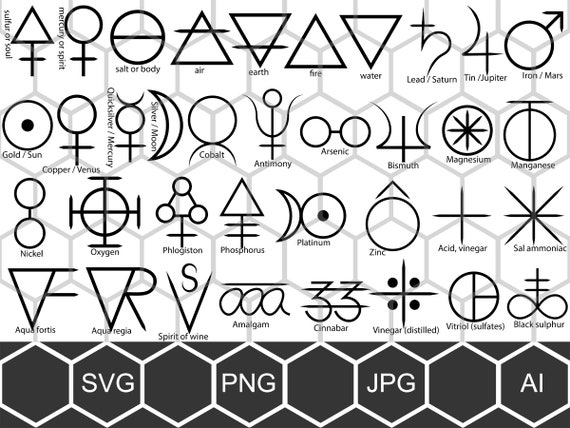This black and white image is a detailed collection of approximately 40 simple line-drawn symbols, likely alchemical in nature, each meticulously labeled with their respective names. The symbols are organized in a grid, set against a light grey honeycomb pattern reminiscent of a bee's hive. Starting from the top left, the labels include "sulfur of soul," "mercury or spirit," "salt or body," "air," "earth," "fire," "water," "lead/Saturn," "tin/Jupiter," and "iron/Mars." The next row features "gold/sun," "copper/Venus," "quicksilver/mercury," "silver/moon," "cobalt," "antimony," "arsenic," "bismuth," "magnesium," and "manganese." Further rows include elements and compounds such as "nickel," "oxygen," "phlogiston," "phosphorus," "platinum," "zinc," "acid/vinegar," "salt," and "ammoniac." The final row presents "aqua fortis," "aqua regia," "spirit of wine," "amalgam," "cinnabar," "vinegar/distilled," "vitriol/sulfates," and "black sulfur." A central feature of the image includes octagonal shapes with labels such as "SVG," "PNG," "JPG," and "AI." This intricate graphical representation intermingles symbols of elements, compounds, and celestial bodies, providing a comprehensive visual summary of alchemical and chemical iconography.